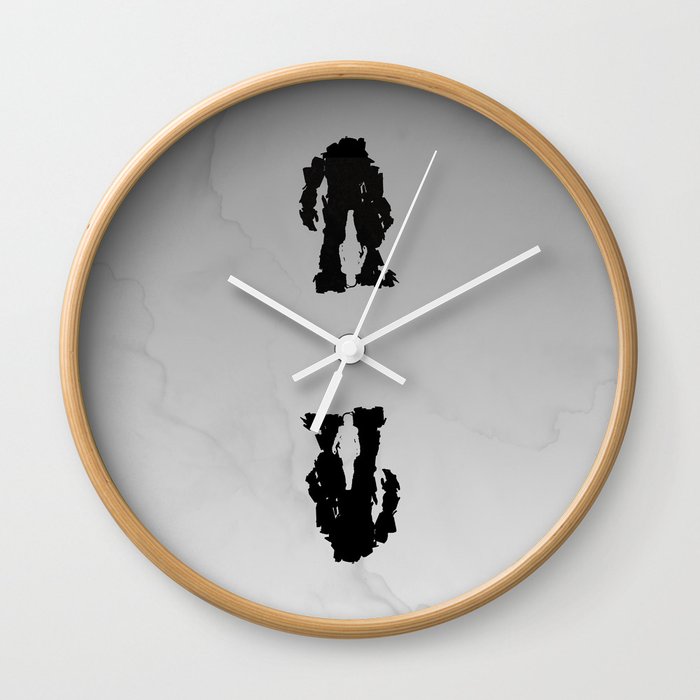In this image, we see a clock set against an off-white background, featuring a wooden circular bezel and a transparent glass face that reveals a cloudy, marble-like grey pattern behind it. The clock does not have any numbers but is equipped with three white hands: a long, thin second hand, a medium-length minute hand, and a shorter hour hand. The time shown is approximately ten past ten, with the second hand indicating a few seconds into the next minute. Embedded within the clock are two mirrored black silhouettes of a power-armored figure. When the figure at the top is right-side up, inside this silhouette is the shadow of a woman walking toward the foreground; the same woman appears upside down within the silhouette at the bottom, which also appears inverted. This complex interplay of shapes and reflections creates an intriguing visual narrative that combines elements of time and motion.